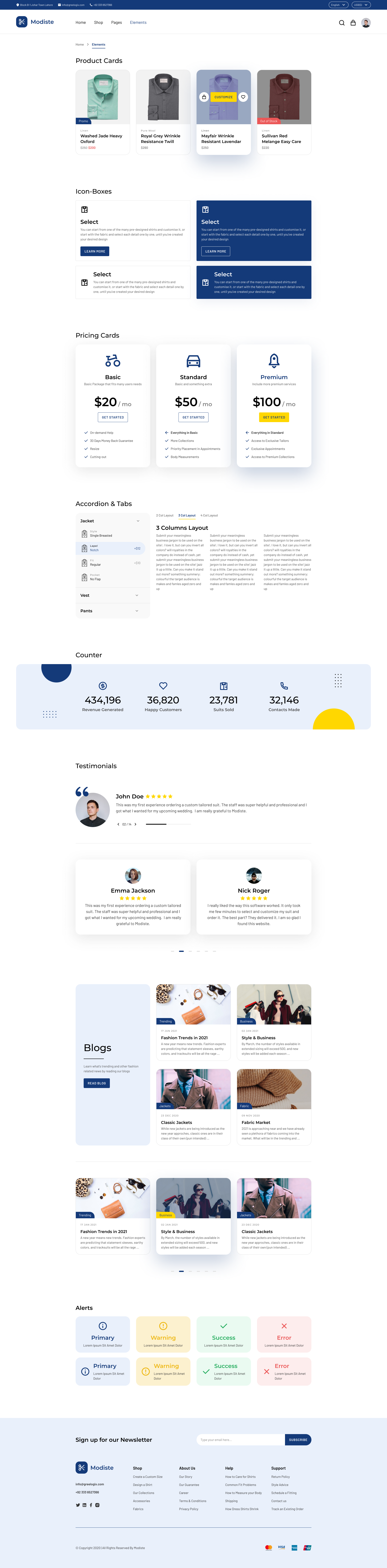**Descriptive Caption:**

A full-length screenshot of a webpage, captured using an app capable of taking extended screenshots, showcases various sections of a website that appears to be selling shirts. The screenshot features a visible horizontal bar at the top, likely the site's header or navigation menu, though the text is too small to decipher clearly.

Below the header is a section displaying four shirts in a single row, each in different colors: teal, dark gray, light purple, and dark orange. The purple shirt is prominently in focus, adorned with three distinct buttons overlaying its image. These buttons include two circular ones with a white background and black text or symbols, and a third button in the middle with a yellow background and black text.

Following the shirts, there's an informational section that likely contains details about the products, potentially including pricing cards labeled as Basic, Standard, and Premium. Another portion of the screenshot appears to contain accordion and tab elements, possibly for organized content display. 

Additionally, there's a section presenting statistical data or performance metrics of the site, accompanied by a large quote and two smaller quotes. The lower part of the screenshot reveals blog entries, with multiple posts displayed. At the very bottom, the page concludes with an area labeled "alerts" and a footer, which typically includes supplementary information or navigation links related to the website.